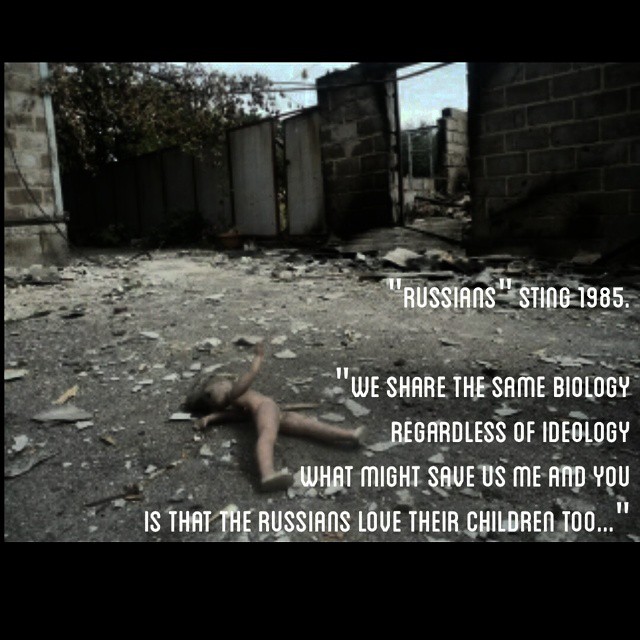The image depicts a desolate, war-torn scene, likely set outdoors. Dominating the bottom half of the image is a crumbling concrete floor littered with debris, possibly from an explosion or some other form of destruction. A weathered, naked baby doll lies amidst this rubble, adding an element of human poignancy to the desolation. The upper half features a dilapidated structure, including a partially destroyed brick wall on the right side, fragments of walls on the left, and what appears to be remnants of a doorway in the middle. The sky visible through the gaps is overcast, contributing to the scene's somber mood. Branches from nearby trees with green leaves hang overhead, contrasting with the grayness of the concrete and the red of the brick. Notably, white text on a black background overlays the top of the image, reading: "Russians, Sting, 1985. We share the same biology regardless of ideology. What might save us, me and you, is that the Russians love their children too." The photograph seems to be part of an awareness campaign highlighting the shared humanity amidst the atrocities of conflict.